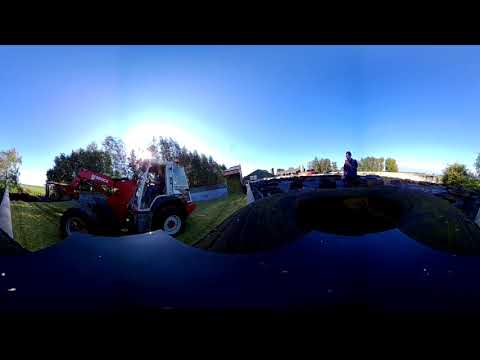This is a small, horizontal rectangular image, dominated by dark tones and a variety of indistinguishable elements due to the overall darkness. At the top of the image, a band of black transitions into a light blue sky that stretches across the upper half. The bottom third of the image is a dark, shadowy area where land or possibly a surface lies, though it's nearly impossible to discern any details in this portion.

In the center-right, a person stands, somewhat lost in the shadow, possibly adorned with sunglasses and black hair, and wearing a dark shirt. Adjacent to this figure, slightly to the left, is a red and white front-end loader or tractor, potentially used for lawn maintenance. This vehicle stands out more distinctly against the otherwise obscured surroundings. Further left, there's a white building or structure and an additional hint of something red that remains ambiguous. This could be a continuation of the vehicle or another structure. 

Echoing across the far left is another white building, perhaps bordering what might be a street or driveway, though the illumination is too poor to confirm. Flanking the center is a line of trees, providing a natural border that seems to stretch uphill, enhancing the feeling of depth and distance. Overall, this scene likely captures a yard or driveway area under maintenance activities, set against a backdrop of clear blue skies.